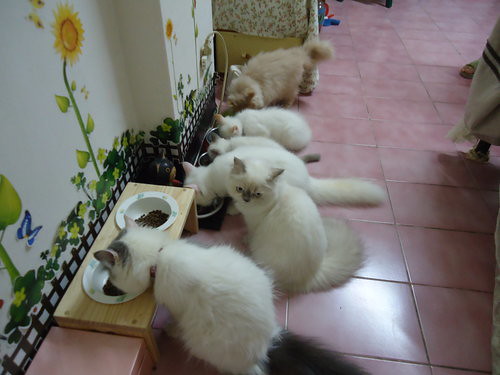In this detailed image, we observe a group of six or seven cats, predominantly white, gathered on a pink tiled floor in what seems to be a room in a house. Among them, a Persian cat with a whitish-beige coat stands out. All the cats are of a similar small size and are eating from individual bowls, which are either metal or porcelain. The cats are aligned close to each other in front of a white wall adorned with sunflower and vine paintings. One cat is curiously looking at the camera, while the others focus on their bowls filled with food.

In the background, a table and a person's sandal-clad foot are partially visible, hinting at human activity within the room. Some small stools with bowls lie in front of the decorated wall, completing the serene yet lively scene of these feline friends.